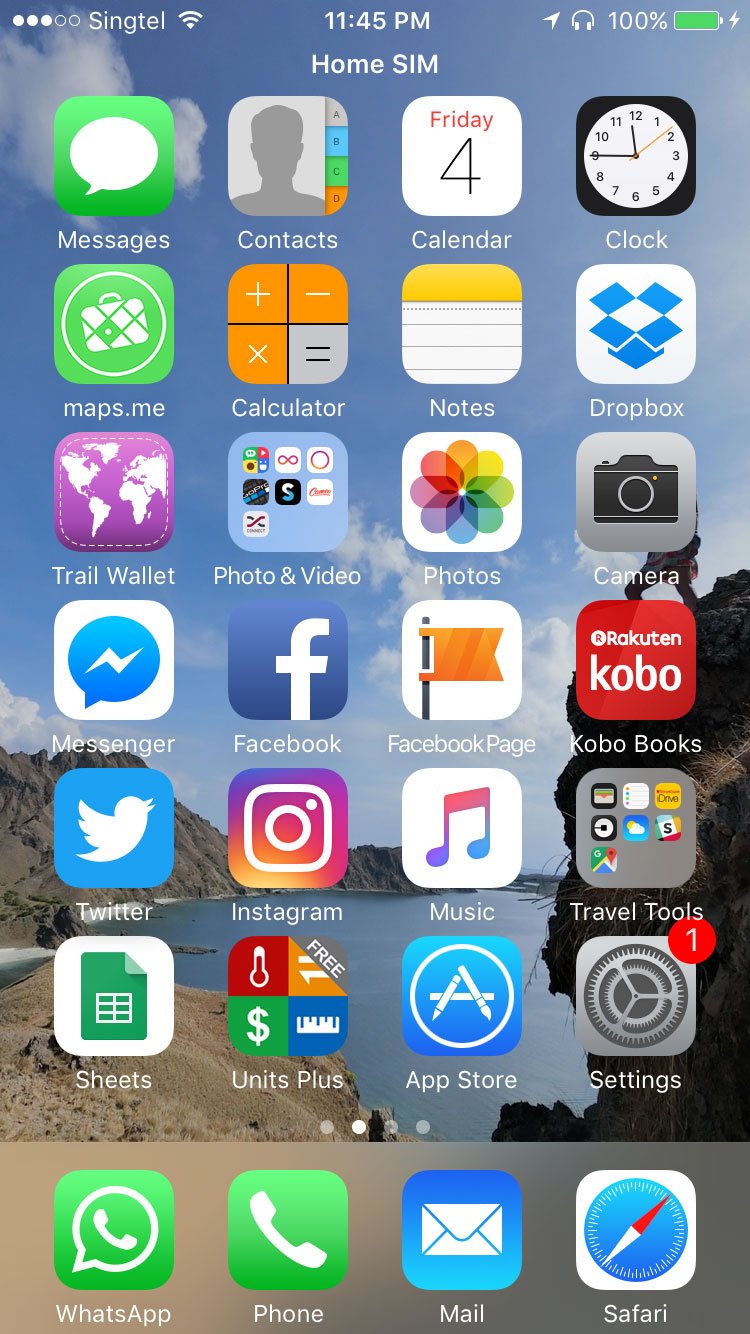In the top left corner of the image, there are three solid dots followed by two hollow dots. Next, there is a Wi-Fi symbol indicating a strong signal. The time displayed is 11:45 PM. A location services icon suggests that location tracking is active. Below these, a headphone icon is shown beside a battery percentage of 100%, displayed in a large green battery graphic.

On the home screen, various app icons are visible. Starting from the top left, there's a green square and a speech bubble representing messages. Next to it, the "Contacts" and "Calendar" apps are displayed, with the calendar showing the date as "Friday 4." Below these, the clock icon, maps app, calculator, notes, notepad, and Dropbox are arranged. Dropbox appears as an open box symbol.

Continuing to the right, a purple icon that looks like an atlas, labeled "Trail One," is present. This is followed by icons for "Photos," showing various colorful images, and "Camera." Social media apps like Messenger, Facebook, Kobo Books, Twitter, and Instagram are also shown. Additional folders or apps are labeled "Music," "Travel Tools," and "Cheats."

At the bottom of the screen, there are icons for "Stop," "Start," "Settings," "WhatsApp," "Phone," "Mail," "Safari," and some other miscellaneous icons.

The background image features a serene ocean scene with mountains in the distance.